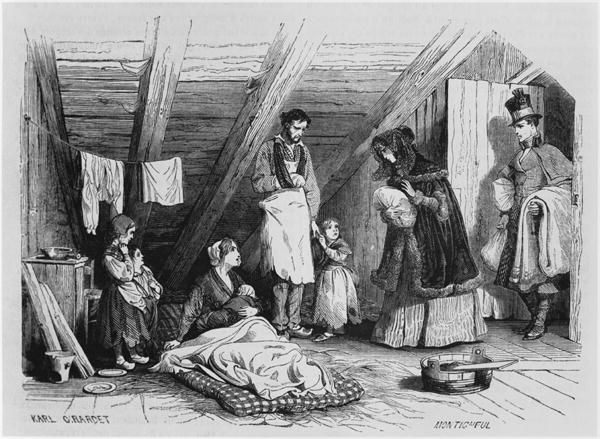This black-and-white illustration, executed in a modern pen-and-ink style reminiscent of woodcuts from the Edwardian era, is set in a humble attic room identifiable by its sloped wooden back wall, visible rafters, and wooden floor. The scene captures a poignant moment involving seven individuals: four adults and three children. In the foreground, a woman with a kerchief on her head is seated on a pallet on the floor, cradling a newborn baby wrapped in a blanket. Surrounding her are two toddlers—one boy and one slightly taller girl—standing close by. 

To her right, her presumed husband, identifiable by his arm in a sling, gently holds the hand of another toddler girl dressed in a long dress and shawl. Above them, two pieces of laundry hang on a clothesline stretched across the attic, adding to the intimate atmosphere. 

The right side of the image features a doorway through which a man in a top hat, outdoor coat, and boots is entering. He carries heavy blankets in his arms. Accompanying him is a woman adorned in a luxurious fur-trimmed hooded coat and a long dress, carrying a parcel. Their attire and demeanor suggest they are of a higher social class than the family occupying the attic. 

Additional details include a wooden bucket on the floor and a small piece of furniture against the left wall. The sketch is signed "Carl Hardett" (or possibly Carl C. Rarset) at the bottom left of the image, with an illegible portion of black font at the bottom right. Four beams run across the ceiling, completing the rustic setting of this evocative attic scene.